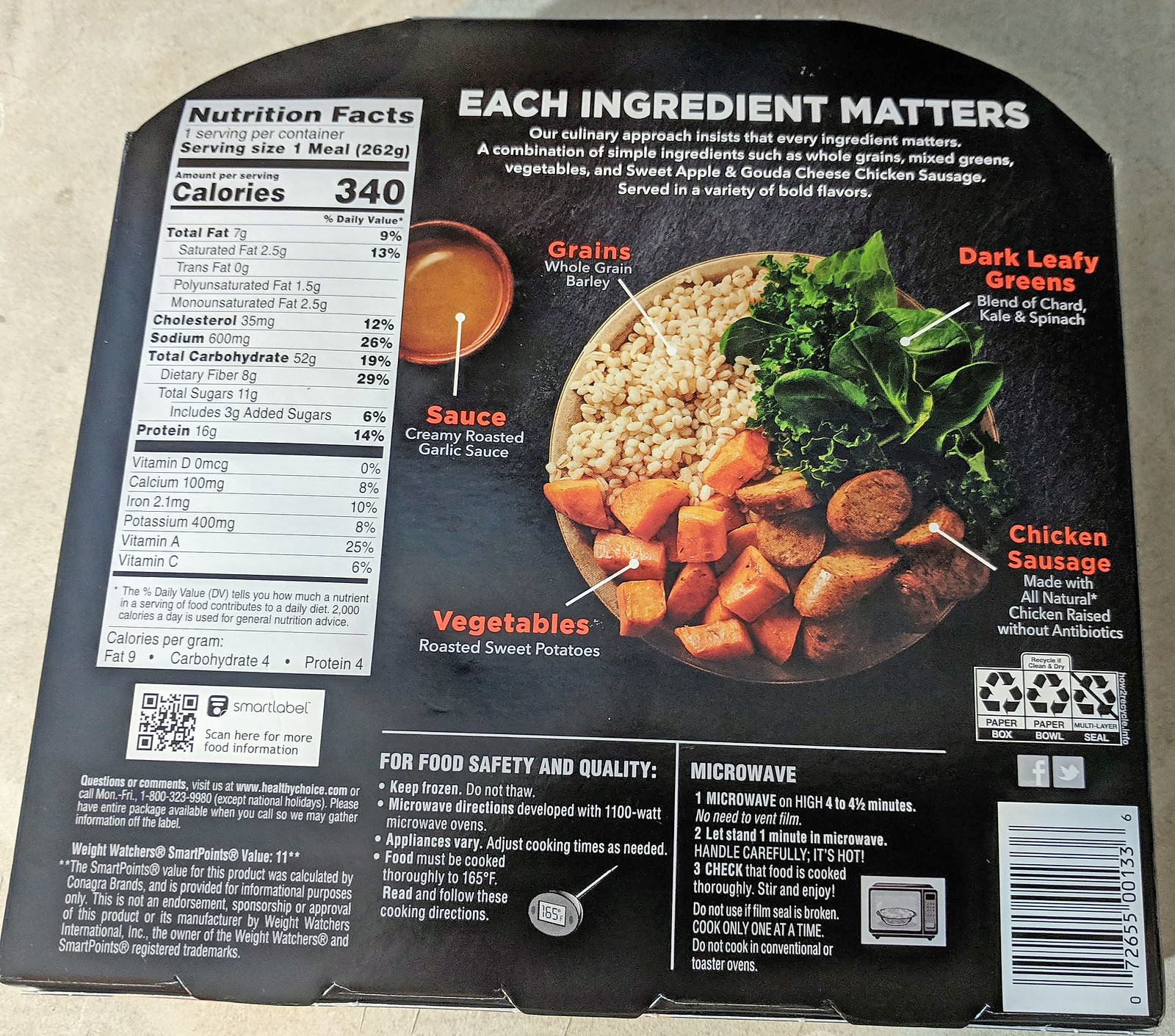This is a photograph of the back of a TV dinner box with a black cardboard background that is mostly square-shaped with a slightly rounded top edge. The packaging features a detailed and informative design. At the top, white text reads "Each ingredient matters. Our culinary approach insists that every ingredient matters." Central to the image is a plate of food, with several components labeled by orange and white text and lines connecting to each item. The labels indicate "whole grain barley" on the left side, "dark leafy greens" (a blend of chard, kale, and spinach) to the right, "chicken sausage made with all-natural chicken raised without antibiotics" at the bottom right, and "roasted sweet potatoes" at the bottom left. Additionally, there is a bowl of creamy roasted garlic sauce located to the upper left of the plate.

To the left of the plate image, nutritional information is provided, detailing calories, total fat, cholesterol, sodium, total carbohydrates, and protein content. Below this section, there are important instructions for food safety and quality, emphasizing to keep the product frozen, not to thaw it, and to cook it thoroughly according to the microwave directions provided. The barcode is located in the lower right corner of the packaging. The image seems to be taken on an off-white, light gray surface, such as a countertop.